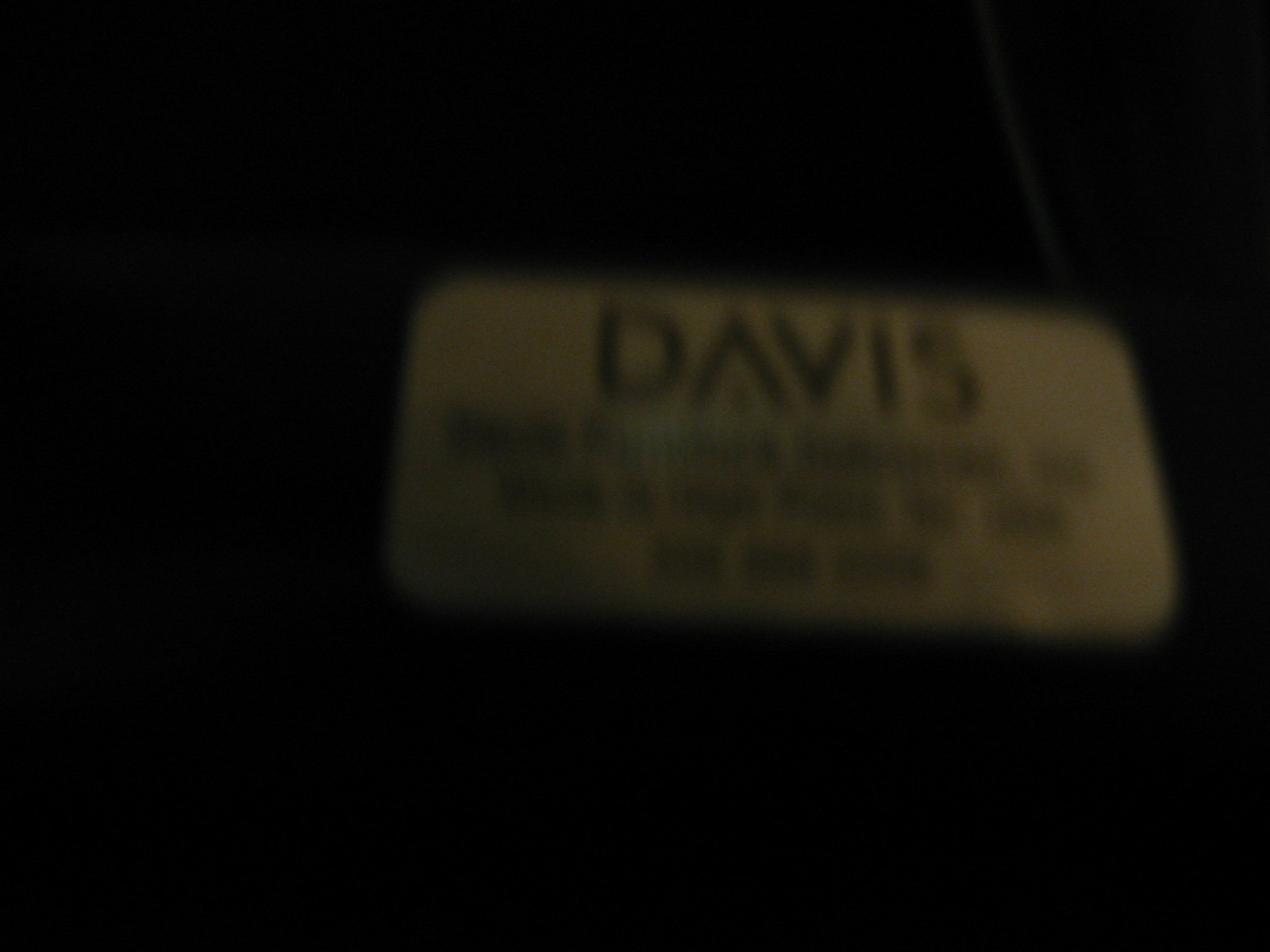A blurry photograph captures a name tag or sign against a pitch-black background. The prominent feature of this mysterious label is a series of partially discernible letters, which appear to spell "Davis." Below this primary line of text, there are three additional lines of much smaller text, though these are too obscured to be legible. The overall effect is enigmatic, with the dark, featureless backdrop adding an air of intrigue to the partially revealed identity.